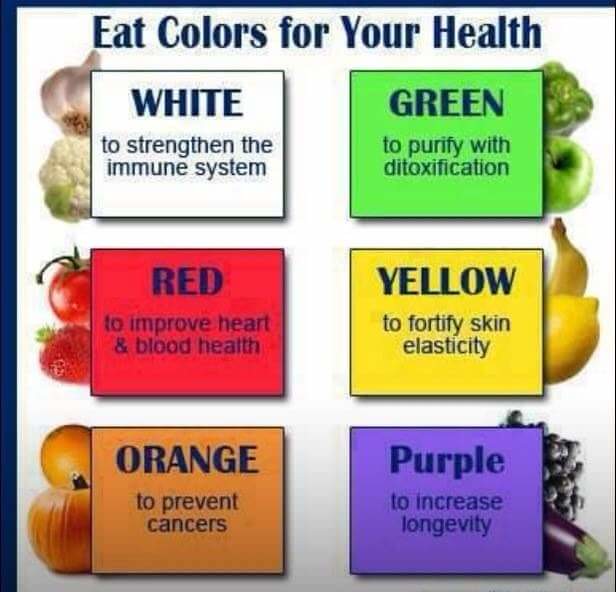The image is an informational poster with a white background, bordered in dark blue, titled "Eat Colors for Your Health" in navy blue at the top. The poster features six vertically aligned squares, three on each side, each representing a different color and its health benefits, all written in navy blue. 

On the left side, the top square is white and is labeled "White to strengthen the immune system," showing images of cauliflower and garlic. Below that, the red square reads "Red to improve heart and blood health," accompanied by pictures of a tomato and a strawberry. The bottom square is orange, labeled "Orange to prevent cancers," and displays a pumpkin and an orange.

On the right side, the top green square says "Green to purify with detoxification," featuring a green apple and a green bell pepper. The yellow square below it states "Yellow to fortify skin elasticity," illustrated by a lemon and a banana. The bottom purple square reads "Purple to increase longevity," with images of an eggplant and grapes. Each square uses corresponding colors to emphasize the health benefits of the featured fruits and vegetables.